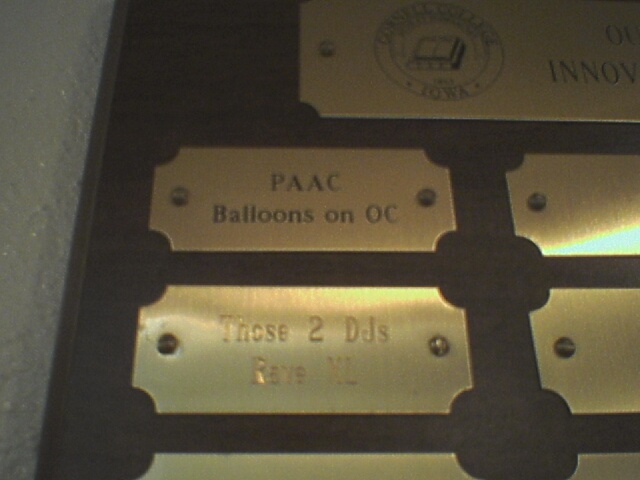The image depicts a close-up of a wooden plaque, set against a white-painted wall. The background of the plaque is made of dark, smooth wood, and it features several brass-colored plates. At the top of the plaque, there is a large golden plate adorned with a circular seal that contains an open book and the word "Iowa" is visible, although partially obstructed. To the right of this seal, the letters "O-V-I-N-N-O-V" are discernible, with the rest cut off.

Below the large plate, on the left-hand side, there is a smaller golden plaque inscribed with "P-A-A-C" and beneath it, the words "balloons on O-C." Adjacent to this plaque, on the right, is another gold plate without any visible writing. Moving further down, on the left, there is another plate that reads "Those Two DJ's" and "Rave N-L." To the right of this, there is an additional plain gold plaque, with no inscriptions. The arrangement and details suggest that the plaques might be honoraries or awards, with some spaces left blank for future inscriptions.